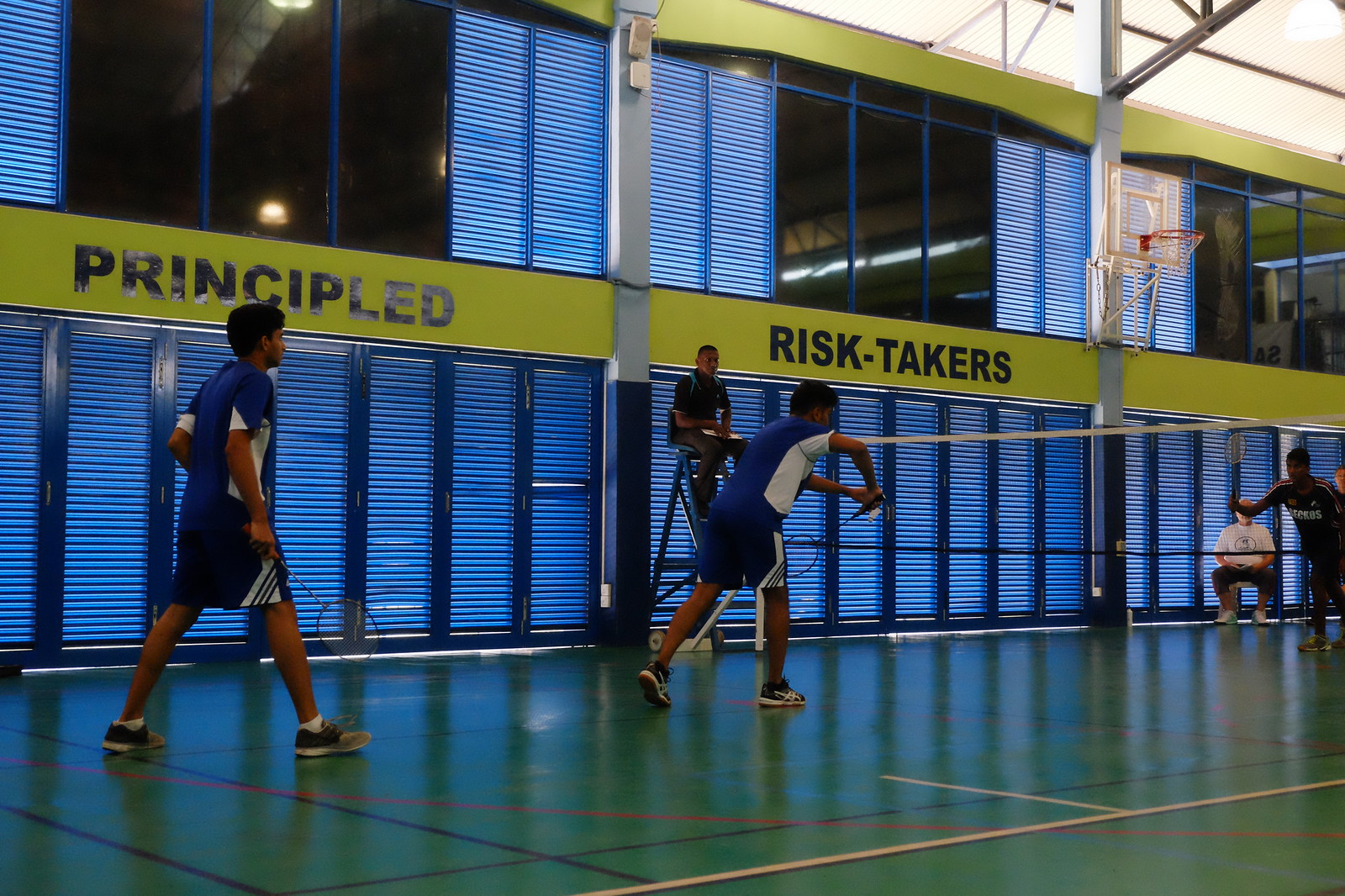This is an action photograph capturing a professional badminton match from the perspective of a corner of the court. The shot is directed towards the court stretching out to the right, with the net placed in the center and extending out of frame to the right. In the foreground, there are two Indian players with darker skin, wearing blue and white shirts and black shorts. The player positioned centrally in the frame is poised to serve the shuttlecock, while his teammate stands nearby. Across the net, an opponent in a red and black jersey holds his racket aloft, ready to respond to the serve. To the side, partially visible, is a line judge wearing a black shirt, seated in an elevated chair near the net. Behind the players, a wall painted in blue, green, and black displays the words "Principled" and "Risk Takers". Adjacent to this text is a white basketball hoop, and seated close to the wall is another individual in a white t-shirt and white sneakers. The dynamic scene is encapsulated within a vibrant and bustling sporting atmosphere.